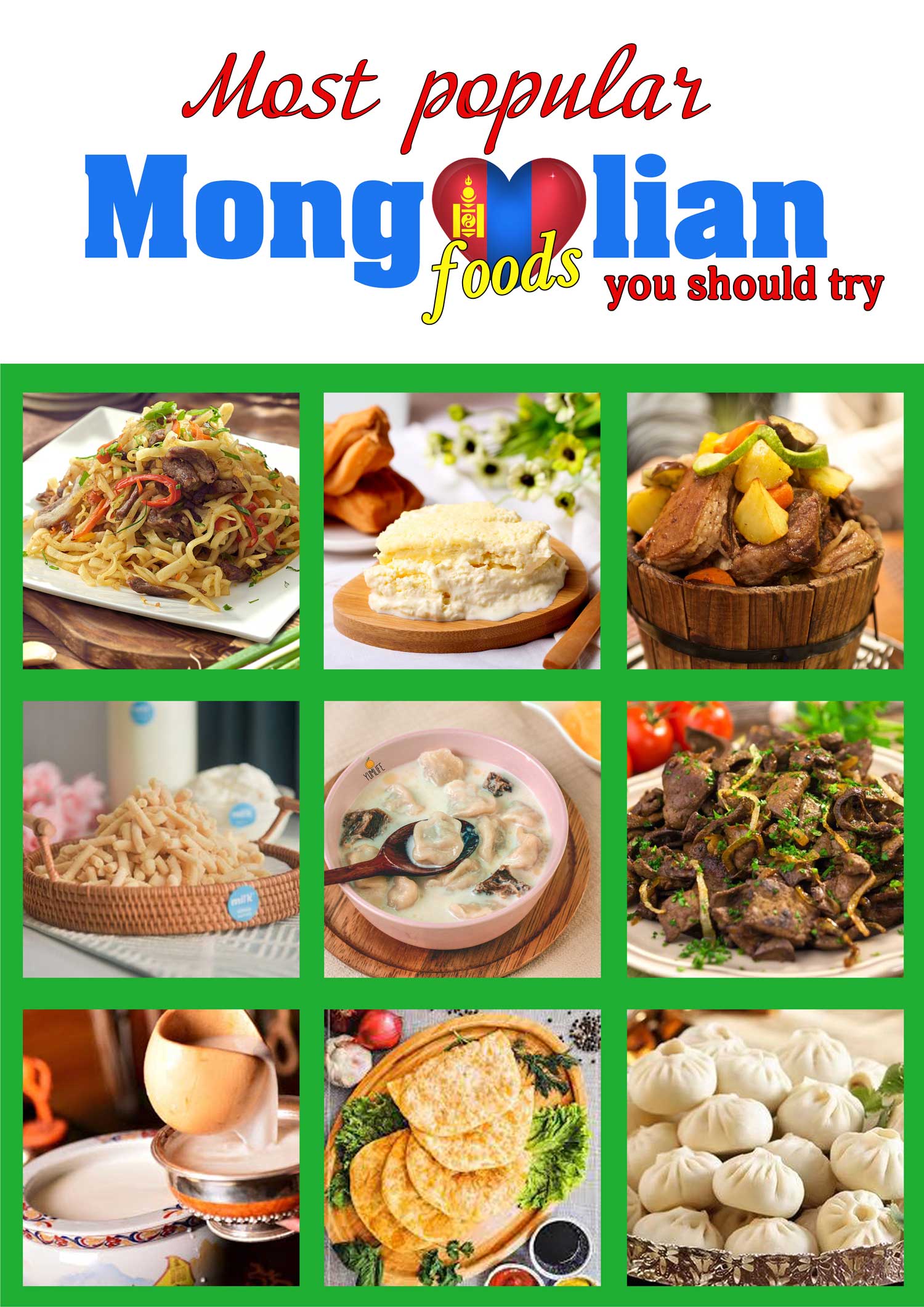The image is an advertisement for a Mongolian restaurant showcasing a diverse range of dishes. At the top of the image, the phrase "Most Popular Mongolian Foods You Should Try" is prominently displayed. The words "Most Popular" are written in red cursive font against a white backdrop. The word "Mongolian" is divided, with "Mong" and "LIN" in blue regular font and a heart shape substituting the second "O," adorned with a design featuring a blue stripe and the word "foods" in yellow at the base of the heart. Completing the phrase, "You Should Try" is also in red font beneath "LIN."

Below this title, a green-framed grid like a tic-tac-toe board displays nine photos, each depicting a different Mongolian dish. The dishes include:

1. Beef and noodles mixture on a white square plate.
2. Pastry or creamy dessert with white cream and cake served on a wooden plate.
3. Potatoes and vegetables, possibly with meat, served in a wooden bucket.
4. Noodle dish presented in a woven basket.
5. Dumpling soup.
6. Mongolian beef dish with noodles.
7. Steamed buns.
8. Bread variety.
9. Milk-based or cheese-based soup.

This menu sign provides a hearty glimpse into the rich and varied cuisine of Mongolia.